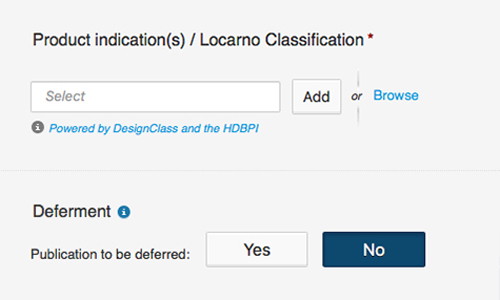Screenshot of a purchasing or product management application displaying a simple, text-based interface on a pale blue background accented with navy blue and aqua print. 

**Page Structure:**
- **Header:** "Product Indication (s)" followed by "Product Indication / Locarno Classification"
- **Input Section:** 
  - A text box (empty) accompanied by an "Add" button.
  - An option divider with "or" between the text box section and a "Browse" link in lighter blue.
- **Information Note:** Below the text box, it mentions, "Info is powered by Design Class and HDBPI".
- **Deferment Section:**
  - A bold heading, "Deferment".
  - Instruction, "Publication to be deferred" in dark, bold text.
  - Yes and No button options, with the "No" option selected in navy blue.

The interface is minimalistic, focused on user input for product classification, offering either manual text entry or browsing options. The deferment of publication can be controlled with straightforward yes/no selections.